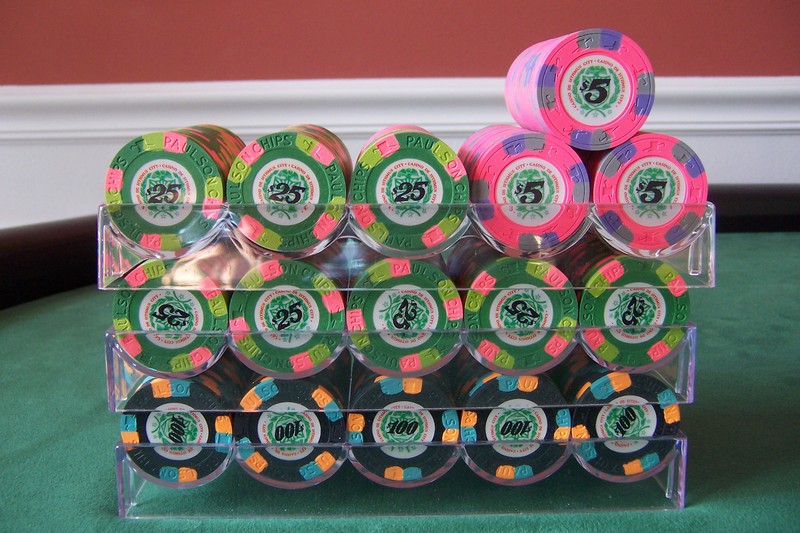This photograph showcases a collection of poker chips organized in three clear plastic trays, stacked atop each other, sitting on a green felt poker table with a dark brown wooden border. The background features a brick-red wall on the top half and a white wall on the bottom, separated by a white chair rail.

The poker chips are neatly arranged on their edges, allowing a clear view of their faces. The top row includes hot pink chips, each adorned with gray and purple squares at the cardinal points and a green center displaying the value of $5. The middle rows contain dark green chips, highlighted with light green and pink squares, marked with the value of $25. At the bottom are black chips, featuring blue and orange squares, and a $100 value at their centers. There are a total of sixteen chips: three rows of five and an additional one balancing on the bottom right row.